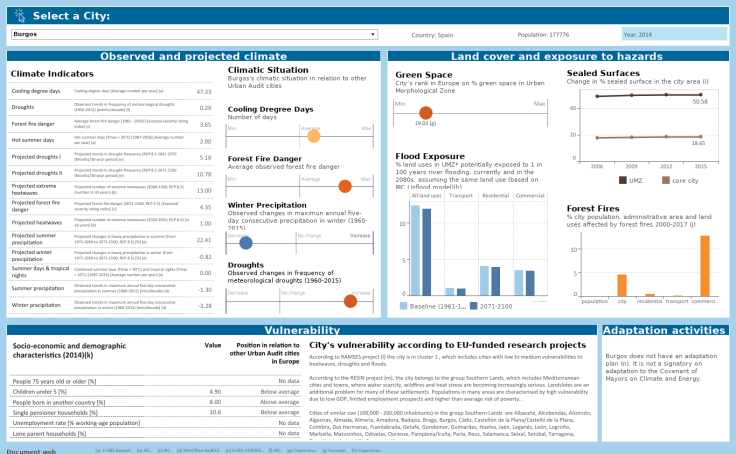The image is a detailed screenshot of a computer screen displaying a sophisticated dashboard with a blue border. At the top, the header reads "Selected City: Burgos," accompanied by a dropdown menu. Below this, there is a section titled "Observed and Projected Climate," featuring various climate indicators such as cooling degree days, droughts, forest fire danger, hot summer days, projected droughts, extreme heat waves, summer and winter precipitation, and tropical nights. The dashboard is filled with a mix of different data visualizations, including line charts, bar graphs, and circular plots. To the right, there is a section for "Land Cover and Exposure to Hazards," while underneath, another section labeled "Vulnerability" details socio-economic and demographic characteristics from 2014, along with the city's position in relation to other urban audit cities in Europe. Finally, on the far right, there is a segment dedicated to "Adaptation Activities." The entire layout is information-heavy and text-dense, potentially overwhelming with the amount of detailed data it presents.